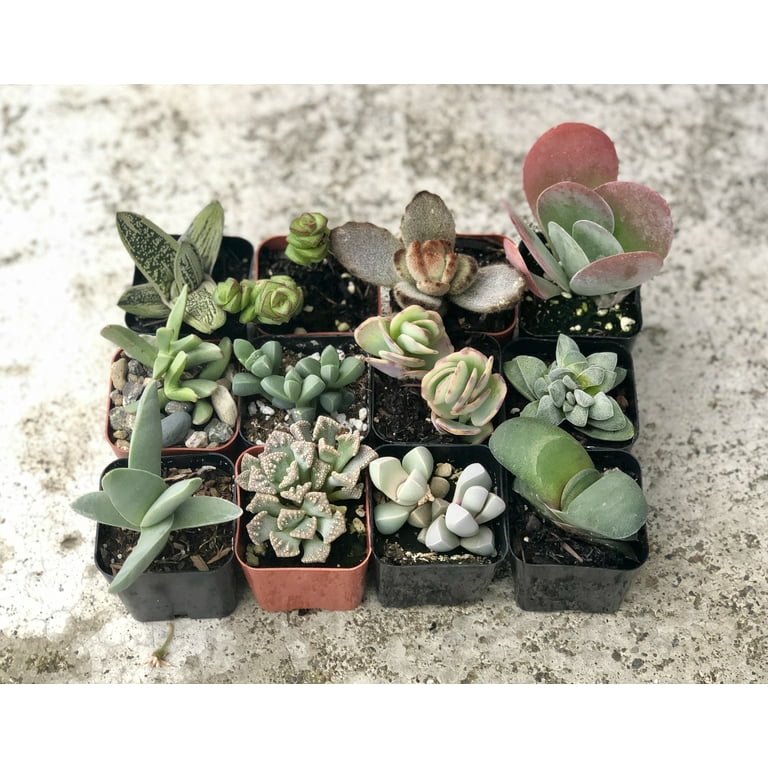The image is an overhead color photograph of twelve small potted cacti and succulent plants, arranged in three rows of four. The pots are square-shaped with rounded corners and sit atop a marble or stone countertop, which is uneven and has a rough texture. There's a distinct lighting effect, with illumination coming from the left, casting the right side in shade.

The plants vary widely in appearance:
- The top left cactus has elongated, oval-shaped leaves with a mottled pattern.
- The top right cactus features large, disk-like leaves that transition from green at the base to red at the tips, resembling a sunrise.
- One of the plants resembles a cauliflower with its intricate, clustered structure.
- Another looks like it’s composed of green cubes.

Each planter contains brown dirt, except for one in the center left, which is filled with small rocks. The plants vary in color from different shades of green to reddish-green, and even pinkish-orange hues. The overall arrangement and variety of the plants create a visually satisfying and detailed composition.